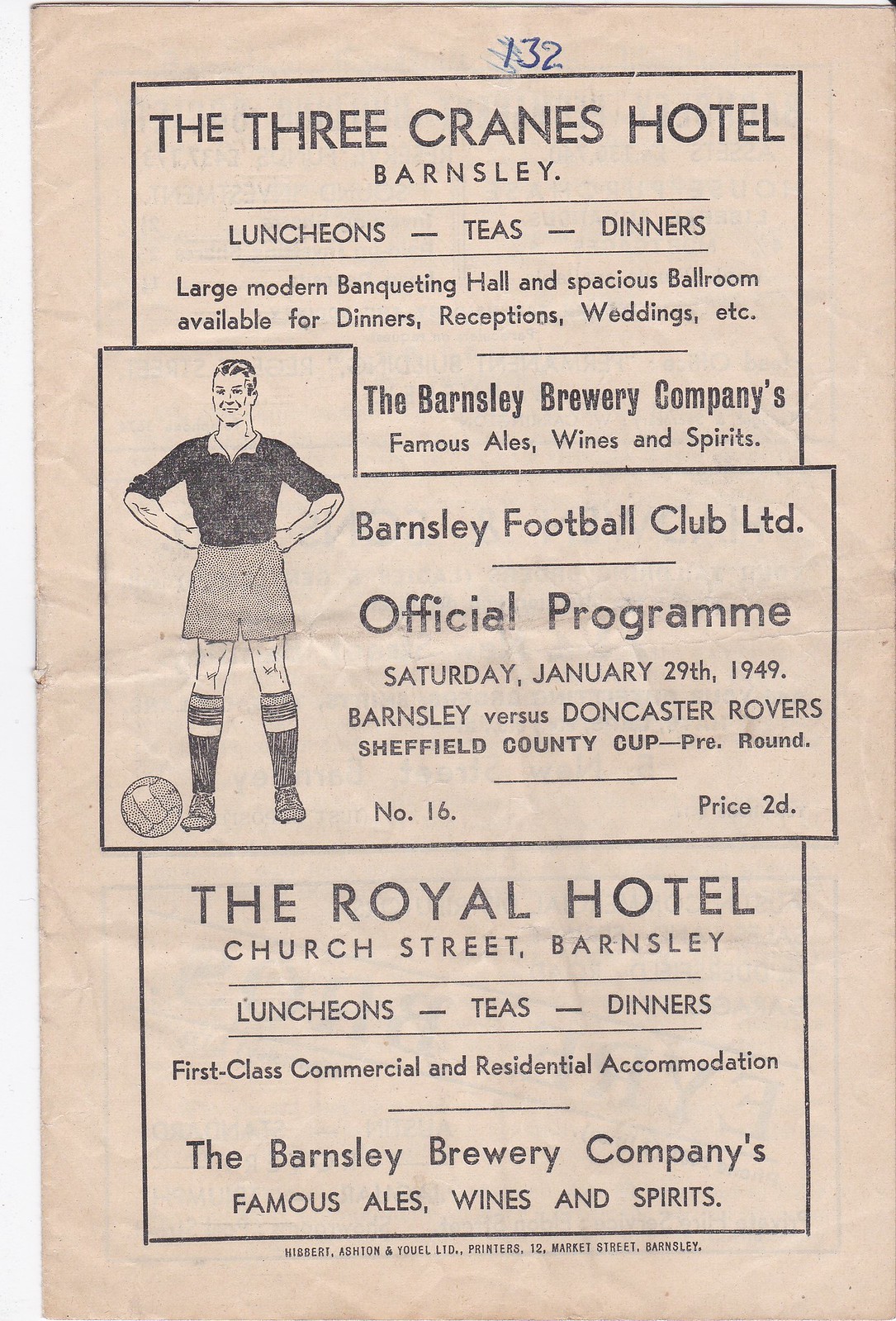This is a detailed, aged pamphlet that appears to be a combination of advertisements and a program page from an old football club. The yellowed paper, which has a noticeable crease in the middle, features the number "132" written at the top in blue ink, though the '1' is somewhat scribbled out, making it appear as "32."

The printed content is organized into three distinct sections. 

At the top, it promotes The Three Cranes Hotel in Barnsley, highlighting its lunch and tea dinners along with a large, modern banquet hall and spacious bathroom available for events like dinners, receptions, and weddings. The advert also mentions the Barnsley Brewery Company's famous ales, wines, and spirits.

In the middle section, framed by an illustration, the content focuses on Barnsley Football Club. It states that this is the official program for a match on Saturday, January 29th, 1949, between Barnsley and Doncaster Rovers, as part of the Sheffield County Cup Pre-Round. This section also notes the program number "16" and the price "2D." The illustration is a sketch of an old-style footballer standing with a round ball next to his foot, hands by his sides, wearing a traditional soccer uniform.

The bottom section advertises The Royal Hotel on Church Street in Barnsley, which also offers lunch, tea, and dinner services. It emphasizes their first-class commercial and residential accommodations, and like the top advert, it also boasts the Barnsley Brewery Company's famous ales, wines, and spirits.

Overall, the pamphlet encapsulates a slice of history with a mix of football culture and commercial advertising, providing a glimpse into the social and sporting life of Barnsley in the late 1940s.